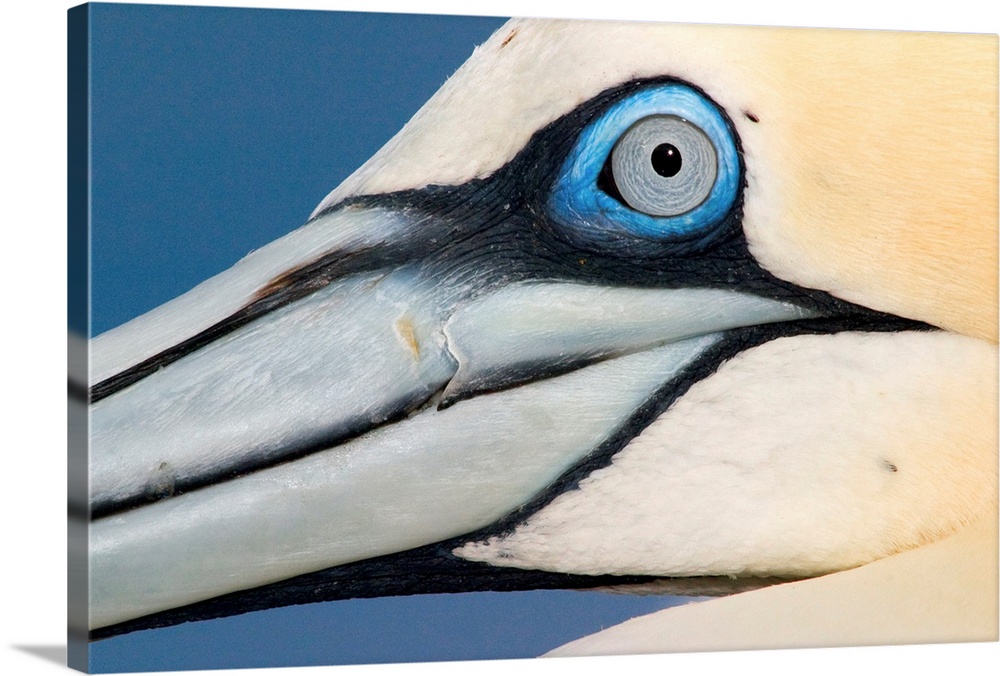This rectangular image, approximately three inches tall by six inches wide, features a close-up, side view of a white bird's head against a deep blue background. The bird dominates the composition with its long, light blue beak extending off the left edge of the canvas. Black stripes accentuate the beak, tracing up to the eye area. The eye itself is intricate, with a black pupil surrounded by a gray inner ring, encompassed by a brilliant light blue outer ring. The majority of the bird's feathers are an ivory or cream color, which slightly darkens towards the upper right-hand corner. A hint of a wing is visible in the lower right-hand corner, adding depth to the painting. Shadowing in the lower left-hand corner suggests that the light source is coming from the right, enhancing the three-dimensionality of the canvas.